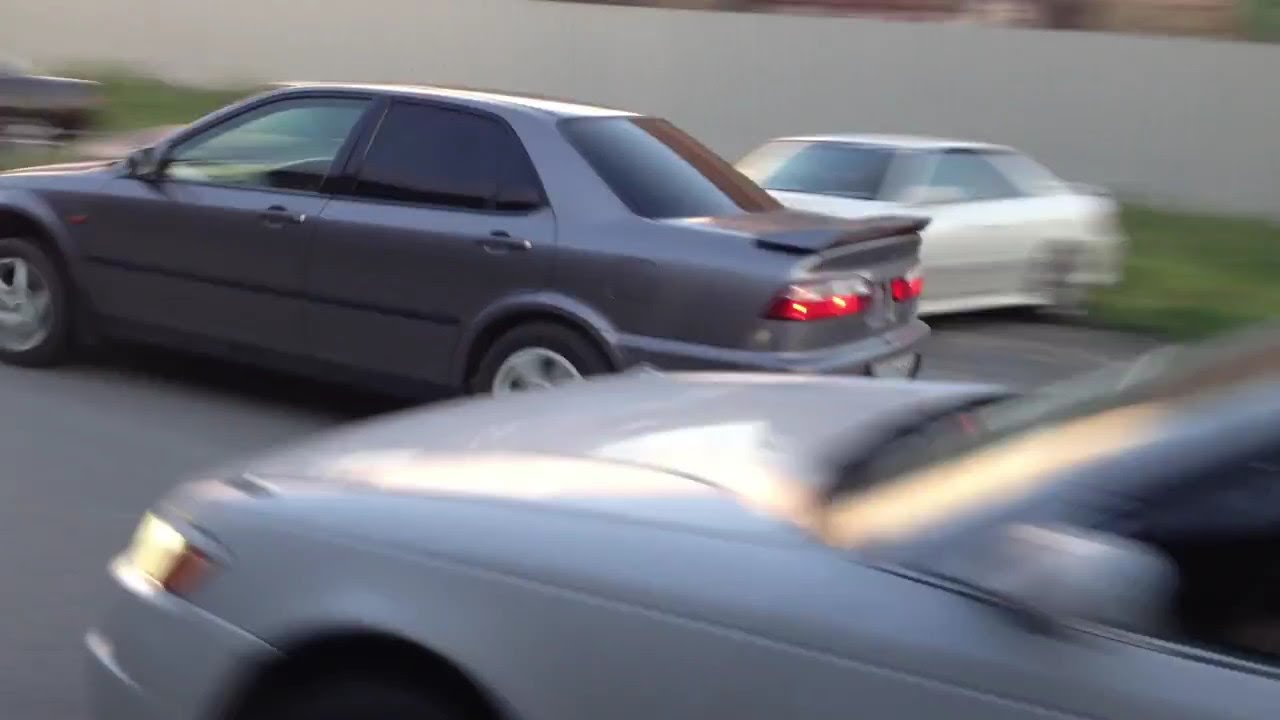The image depicts a dynamic scene with three cars in various states of motion and blur, suggesting they are racing or moving swiftly through the frame. In the foreground, a silver sedan, its headlights beaming, is prominently featured. The vehicle’s front wheel arch, side door, and window are all visible, albeit blurred due to the speed. To its left, a light gray car, almost fully captured in the shot, displays red taillights and a small spoiler, with black-tinted windows marking the rear passenger area; the dashboard and interior plastic components are discernible. In the background, a white two-seater car appears stationary, positioned against a gray wall with a stretch of green grass running along the image's rear. The overall ambiance suggests a movement from right to left, with the scene occurring possibly in the early evening, given the active headlights on the silver car and the taillights on the gray car. The backdrop includes a mix of subdued colors, adding context to the urban or suburban setting.